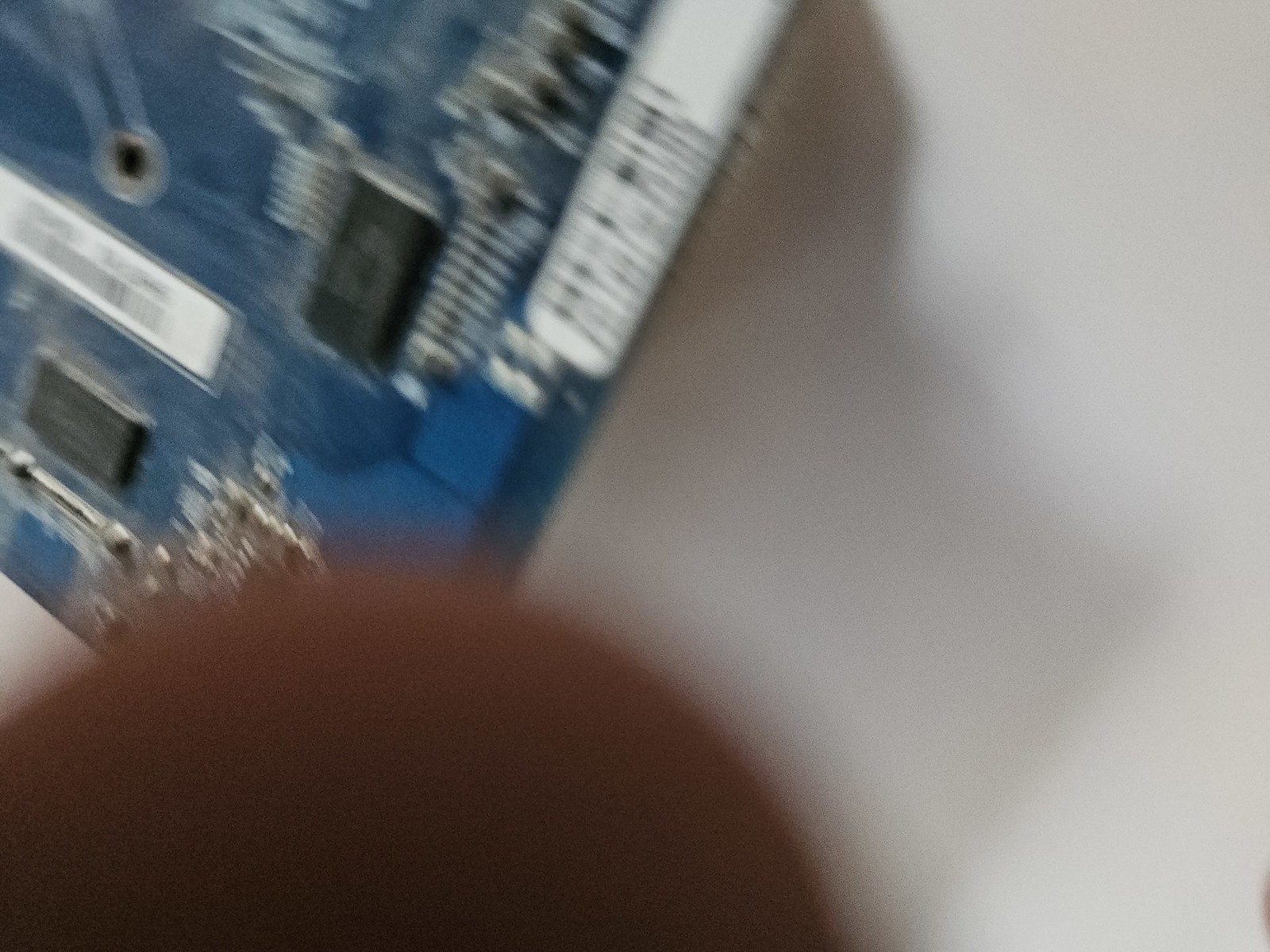This photo captures a very blurry close-up of a corner of a blue electronic motherboard featuring various black components soldered onto it. A finger partially obscures the bottom left of the image. The motherboard is detailed with numerous shiny silver soldered parts and includes white labels: one prominently in the middle-bottom and another on the left side, extending diagonally downward. The background on the right side is white, likely a wall, casting a shadow of the motherboard. There are also scattered silver details and wires, adding to the intricate and somewhat chaotic appearance of the image.